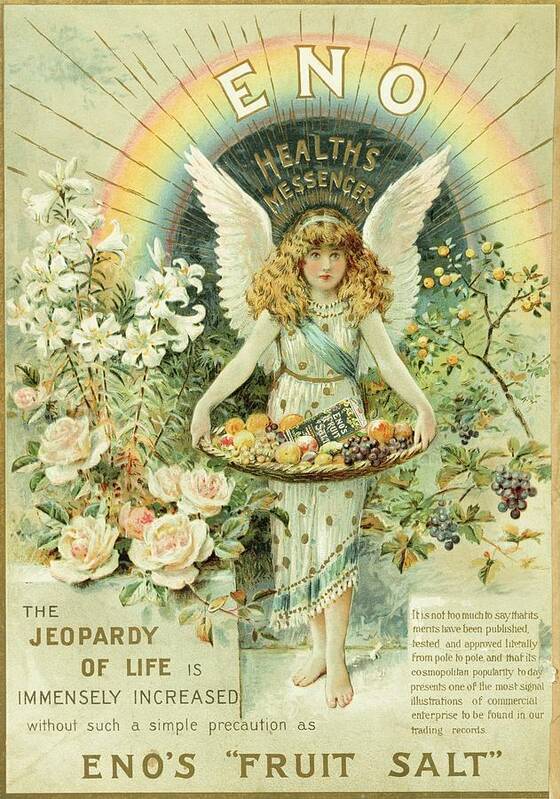This is a vintage advertisement poster resembling early 1900s American art style. The background is a grayish, yellowish, creamy color, with a rainbow arching from the top towards the sides. At the center stands a winged angel with long curly hair flowing past her shoulders, reminiscent of Renaissance art. She wears a greenish-cream dress adorned with gold spots and gold trim, an uneven hem that rises to the right and drops to the left, and a blue sash. She holds a basket filled with various fruits and appears to be about 12 years old. The angel is surrounded by an array of flowers: pink roses, white tulips, and white lilies on the left, along with berries and oranges on branches to the right.

Bold and prominent at the top of the poster is the word "ENO," followed by the tagline "Health Messenger." The bottom of the poster emphasizes the product, Eno's Fruit Salt, with the impactful statement, "The jeopardy of life is immensely increased without such a simple precaution as ENO's fruit salt," printed in bold. Additional text at the bottom right mentions that the product has been "published, tested, and approved literally from pole to pole." The entire poster is bordered in gold, adding an elegant frame to the detailed and colorful advertisement.